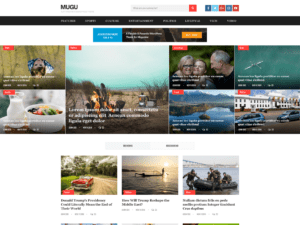The image showcases a blurred web page interface, providing a vague impression of its layout and structure:

At the top left corner of the page, there are discernible black letters "M-U-G-U". Adjacent to these letters on the right, a search bar is visible, though its contents remain indiscernible. Alongside the search bar are several clickable icons, likely representing social media platforms.

Beneath this upper section lies a black navigation bar featuring eight distinct options, labeled in white text that is unreadable due to the blur. Directly below this navigation bar, there is a blue box adjacent to a black box, the latter having an orange insert. Both boxes display white text, which again is illegible.

The main body of the page exhibits ten photographs, each depicting various scenes and activities. Among these, there's imagery suggesting people dining, likely outdoors, and possibly on vacation. One photo appears to showcase a hotel, another a river, while others illustrate dining settings with fruit or salads. Additional images at the bottom left include men in wetsuits kayaking, an old-fashioned red convertible car, and someone on a boat at sundown.